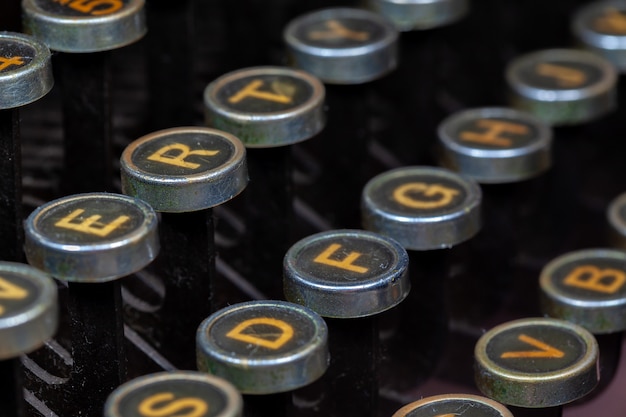The up-close image features an old typewriter, likely from the 1940s or 1950s, with round, silverish keys on a dark gray background lined up in orderly rows. The keys, which are dusty and appear to have not been used in a long time, have letters and numbers in an orangish-yellow color. The letters visible are W, E, R, T, Y in a row, followed by S, D, F, G, H, J, and then V and B below. At the top, parts of the numbers 4 and 5 can be seen. The keys are arranged closely together horizontally while the rows have a bit more space vertically. The background is black, giving the impression that the typewriter is in a container or perhaps just emphasizing the age and disuse of the machine.